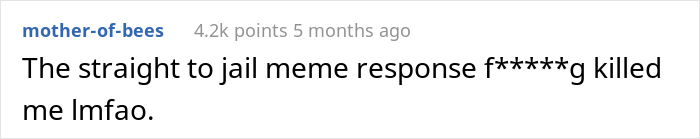The image depicts a single entry on a message stream, framed by a rectangular border with a gray trim. The background inside the rectangle is white, providing a clean backdrop for the content. In the upper left-hand corner of the entry, the username "mother-of-bees" appears in all lowercase letters, colored in a medium blue. To the right of the username, the entry displays "4.2k points," followed by "five months ago" indicating the post's popularity and age.

The main body of text within the entry is in a large black font. It reads: "The straight-to-jail meme response effing killed me" without a period at the end. Below this sentence, an abbreviation "I am FAO" followed by a period is visible, indicating laughter. The overall layout gives a sense of an informal conversation within a social media or forum thread, likely one where users are reacting humorously to shared content.